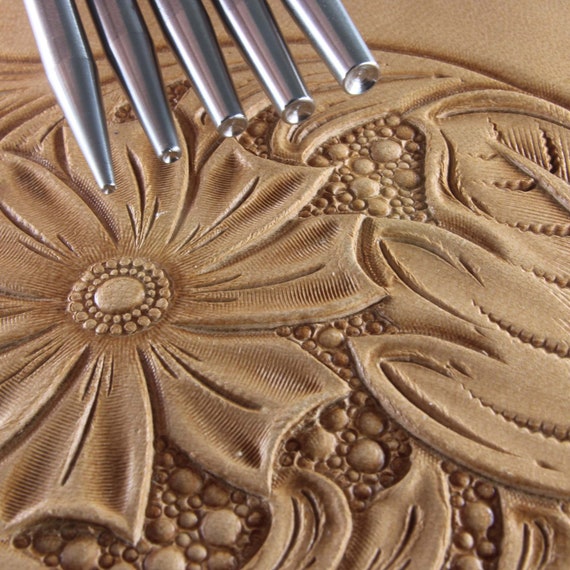The image is a detailed close-up of unfinished or untanned leatherwork, featuring a prominent, intricately crafted flower with large petals and surrounding leaves. The background has a dark sandy color, adding texture and contrast to the floral design. In the upper left corner, five silver metal tools, resembling pens or knitting needles, are arranged in a line, seemingly used in the creation of the design. These tools, varying in size with different tips, are positioned towards the flower, emphasizing the craftsmanship involved. The overall texture and unfinished quality suggest that the leatherwork is a work-in-progress, although there is a possibility that the material could be light-colored wood.